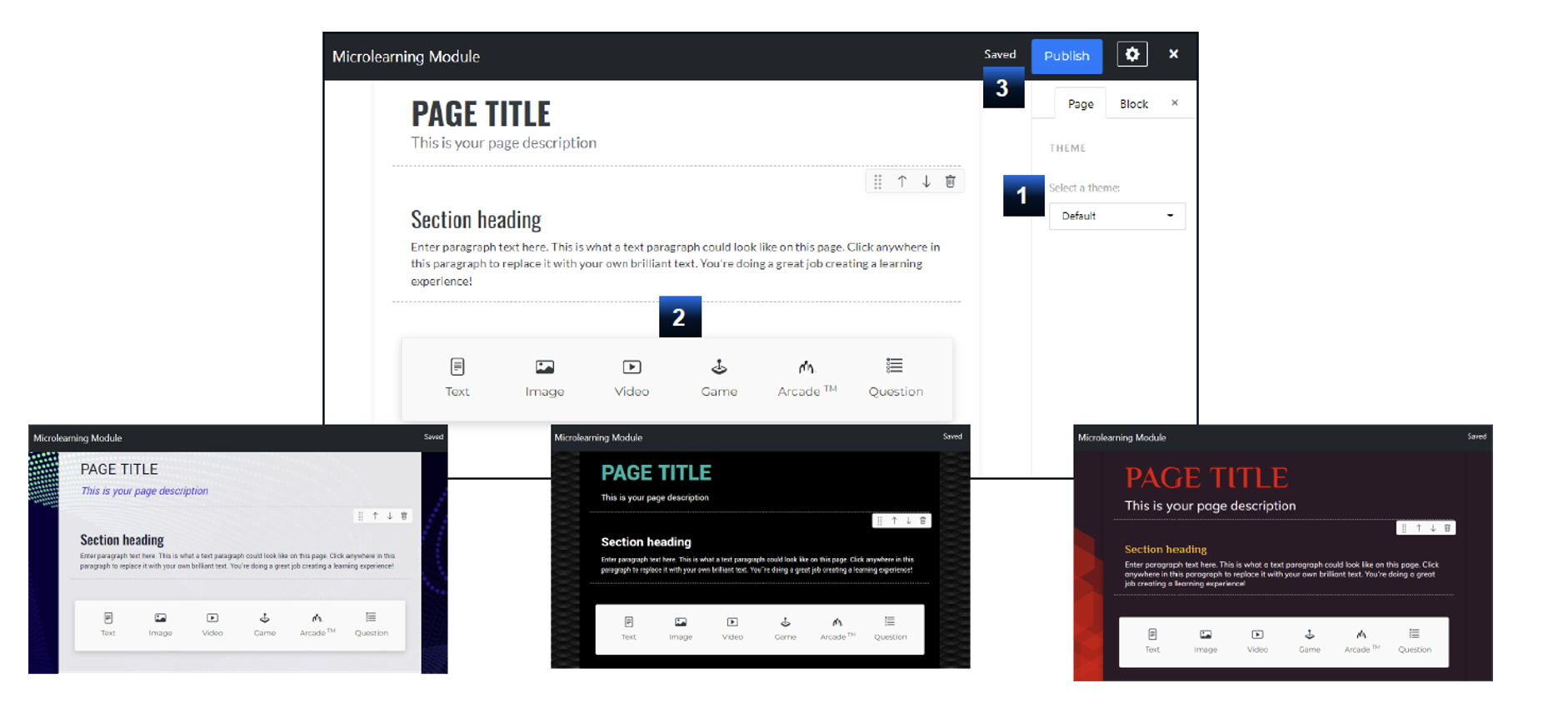The image features a detailed layout with four distinct boxes:

1. **Top Box**: This box is outlined in black. At the top, there is a black header labeled "Micro Learning Module". Next to this label, there is a blue drop-down box displaying the number "3". Adjacent to the drop-down is a blue "Publish" button, followed by a small cog icon and an "X". Below the header, the box has a white background with text areas labeled "Page Title" and "This is your page description". There's a blue box containing the number "1", accompanied by several smaller boxes with arrows. Further down, there is another section called "Section Heading", which includes a blue box with the number "2" and several icons at the bottom.

2. **Second Box**: Outlined in dark blue, this box has a little fingerprint icon situated in the top left corner, along with some white print. Inside, there is a light blue box featuring "Page Title" and "Section Heading". Below, a small white box contains various icons.

3. **Third Box**: This box has a black background with small white text at the top and on the right-hand side. Within the black background, a green "Page Title" stands out, followed by a small white box, another heading, and a large white box at the bottom containing several icons.

4. **Bottom Box**: This box combines black and red elements, featuring red cloud-like shapes on the left side. White text is placed at the top, and a red "Page Title" is followed by the text "This is your page description". The box also includes a smaller box with red and white print, along with a white box depicting several icons.

Each box is intricately detailed with various labels, buttons, icons, and color-coded sections, forming a structured and comprehensive layout.